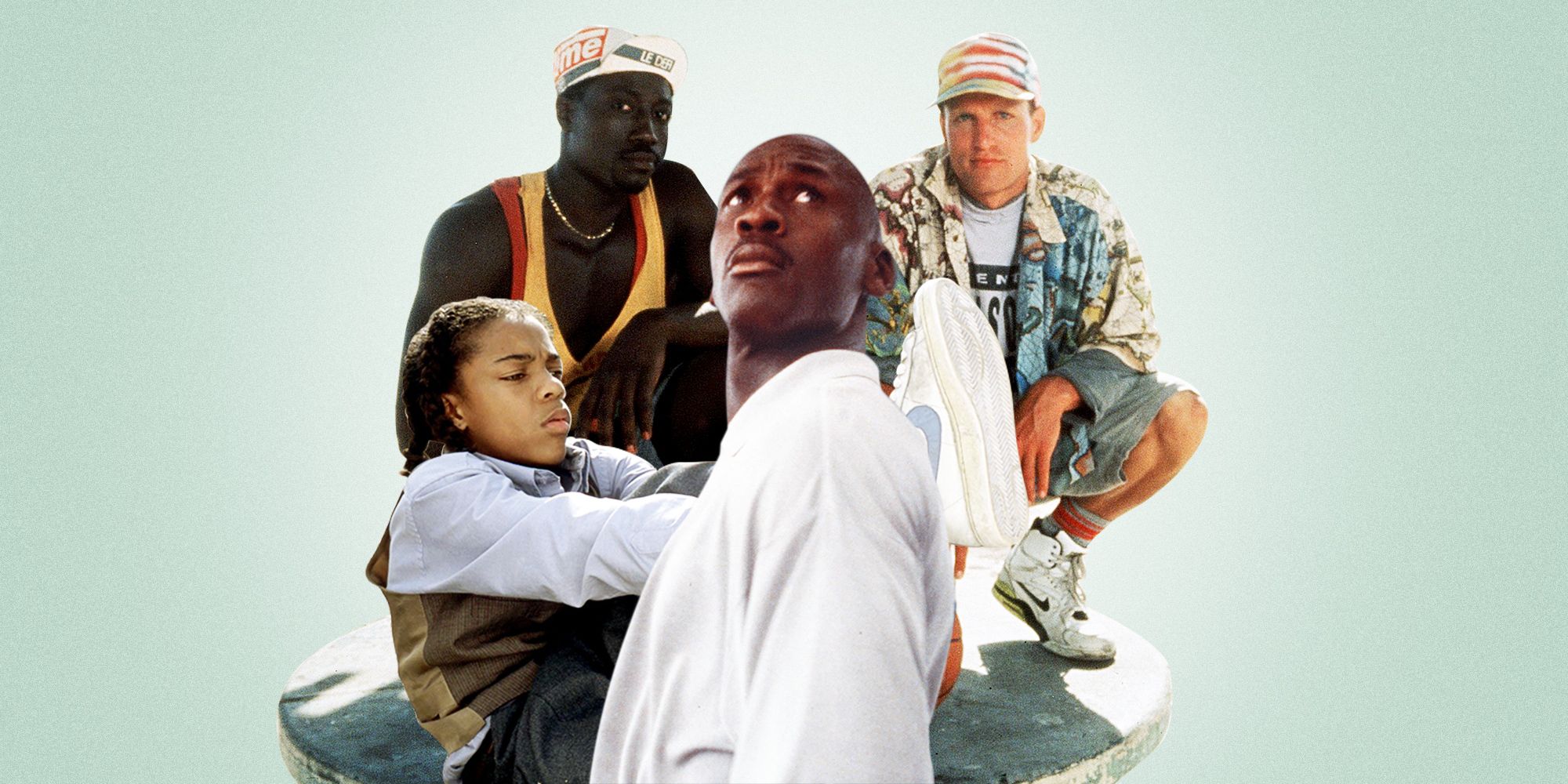In this composite or potentially collaged image inspired by the movie "White Men Can't Jump," four individuals are displayed against a gradient greenish-blue backdrop that darkens towards the edges with a bright center. Dominating the foreground is an African American male, likely in his thirties, with a balding head and a slight mustache. He sports a long-sleeved white shirt and is captured from mid-waist up, gazing upward and to the right, his arms hanging loosely by his sides.

Behind him squats a white male, also approximately thirty years old. His muscular calves are accentuated by his blue denim shorts, which reach his knees. He wears high-top white Nike sneakers with a black swoosh and a long-sleeved plaid shirt. His left elbow rests on his upper thigh, and his wrist dangles down. A red, white, and greenish-blue striped baseball cap adorns his head. This individual, likely representing Woody Harrelson, looks straight into the camera with a serious expression.

To the right of this white male and slightly back is another African American man with dark brown skin and a gold chain around his neck. His head, featuring a serious expression, is turned slightly to the right, showing only his left ear. He’s donned in a mostly white cap with black and red lettering, along with a yellow and red vest over a bare chest, resembling Wesley Snipes’ character from the movie.

Lastly, seated on a round concrete or pale platform, facing slightly to the viewer's right, is a young girl, seemingly around twelve years old. Of mixed African-American and European-American descent, she has light brown skin and a serious expression with partially shut eyes due to sunlight. She wears a white top, possibly a tan vest, and dark shorts, with her arms extended out in front of her.

All individuals in the image share a solemn demeanor, creating a distinct contrast against the playful reference to "White Men Can't Jump."